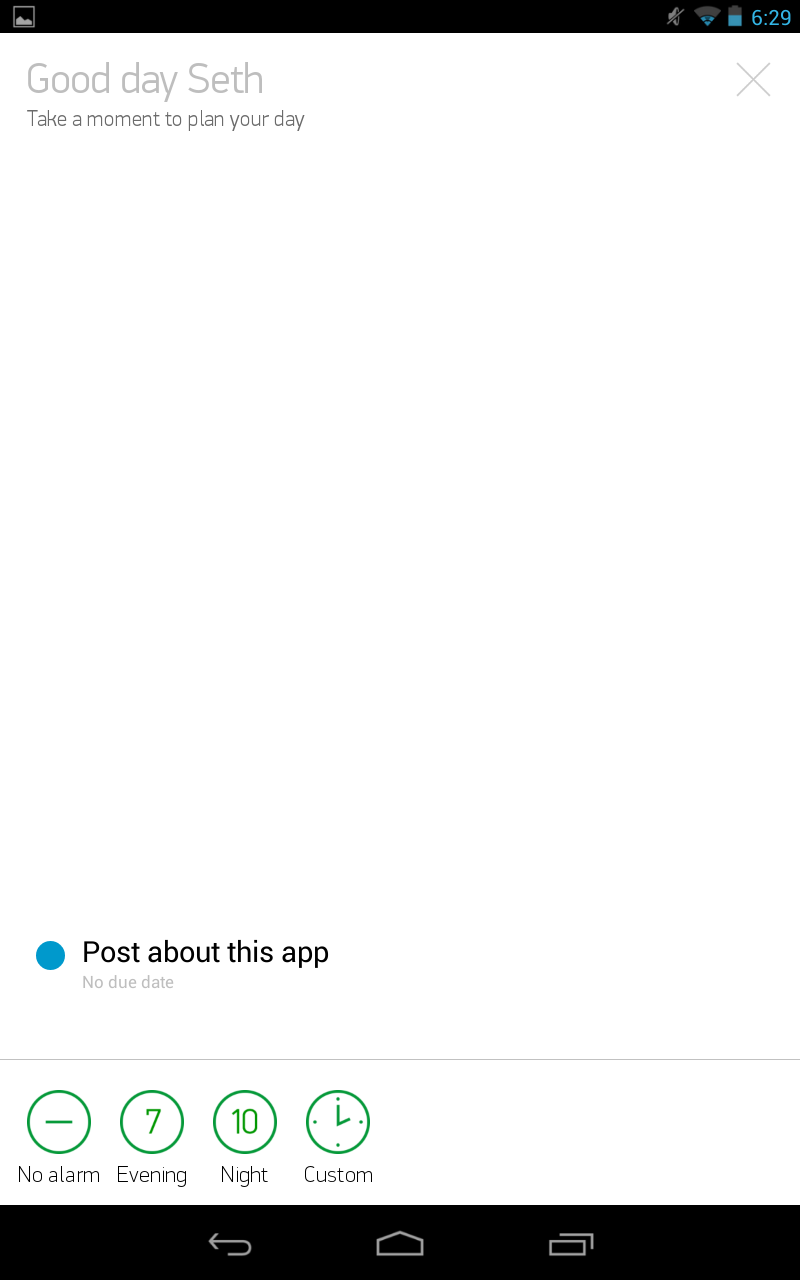Screenshot of a cell phone interface with productivity features:

The image is a screenshot of a cell phone screen, devoid of any background and showcasing the interface of a productivity app. The rectangular shape of the phone is inferred from a thin black horizontal bar at the top and a taller black horizontal bar at the bottom.

At the top bar, the screen displays essential status icons - the time indicated as 6:29, alongside a battery icon and signal strength indicator. On the left side of the top section, gray text greets the user with "Good day, Seth," followed by a smaller caption, "Take a moment to plan your day." An 'X' icon on the right side likely allows users to dismiss this greeting and message.

The screen predominantly appears blank, except for a notable blue circle button at the bottom with the text, "Post about this app. No due date." Just below this button, a thin, light gray horizontal line separates it from a series of green circles. These green icons are labeled "No alarm," "Evening," "Night," and "Custom," suggesting different time-related settings or reminders.

Anchoring the bottom edge of the screen, within the black bar, are three icons hinting at navigational or functional buttons related to the app’s core features. These elements suggest that the app is designed for organizing and planning daily activities, likely synced with a calendar, habit tracker, or to-do list focusing on time management and productivity.